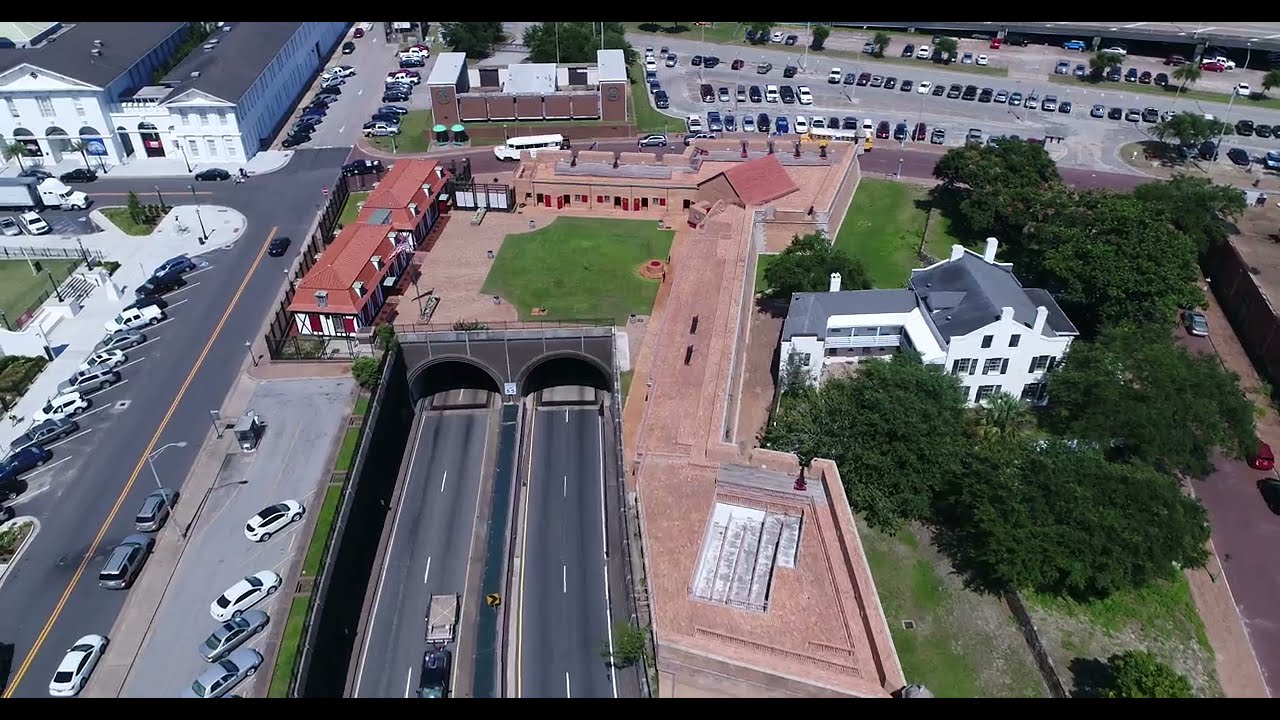This overhead photograph captures a vibrant downtown area, possibly an office park. The scene is dominated by several commercial buildings, among which a distinctive, long brick building with multiple sections stands out. Close to this building, a large white structure with a red roof is noted, surrounded by an expansive red brick walkway. Adjacent to it, another white building with a gray roof is visible, encircled by thick green trees and grassy areas. Throughout the image, numerous parking lots are filled with parked cars and trucks, highlighting the area's bustling activity. There is a prominent road network with visible traffic, including a freeway that creates an underpass beneath the large red platform. A diesel truck and several cars are seen moving through this tunnel. The right and left corners of the image reveal additional large white buildings and more parking spaces. The overall scenery suggests a sunny day, with observable shadows cast by vehicles and structures, and while there are plenty of vehicles and traffic, human presence is not directly visible.